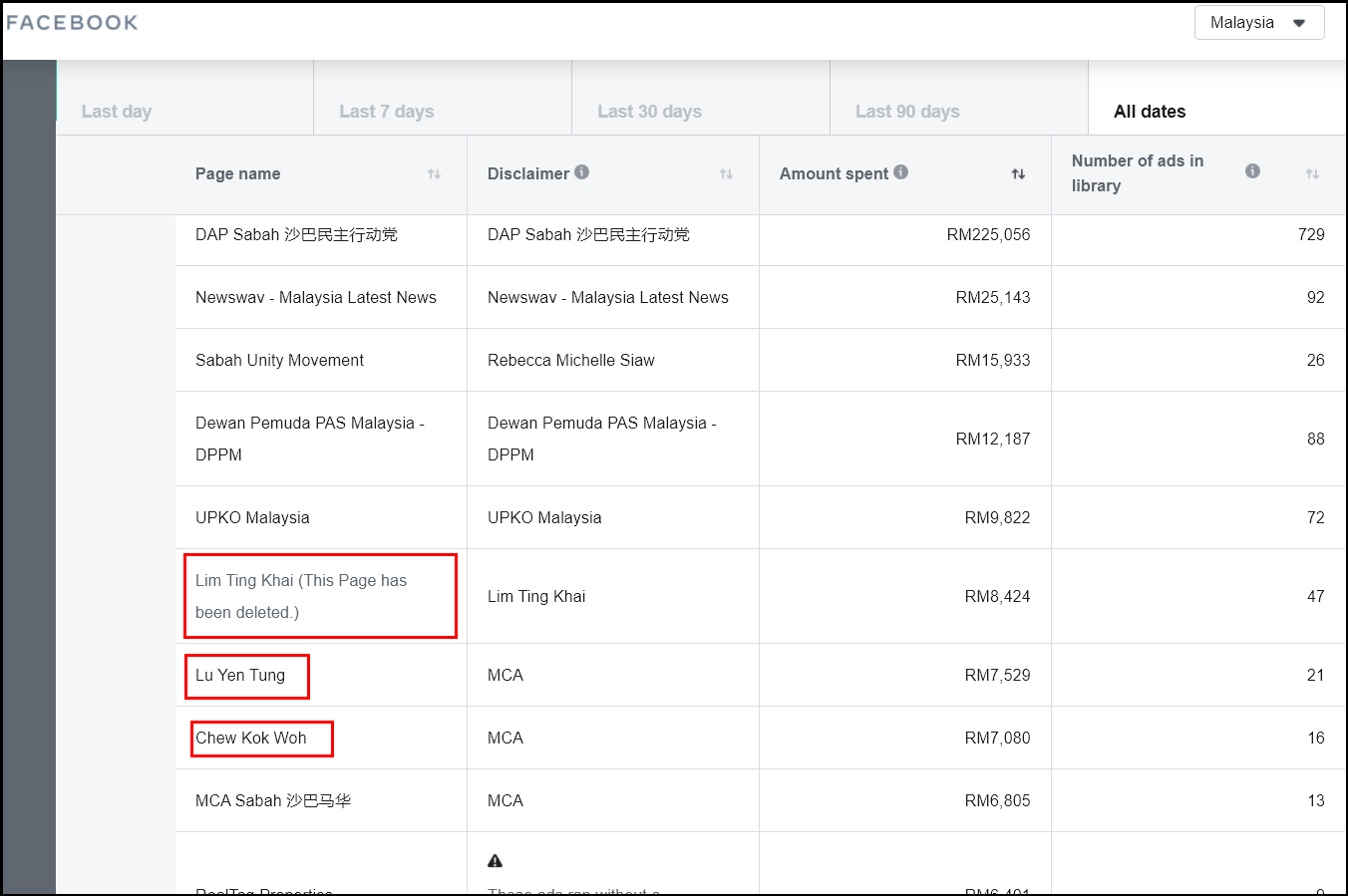A detailed depiction of the image:

This image features a predominantly white square background with various informational boxes. At the very top center, there's a small white box labeled 'Facebook' in gray text aligned to the left. Below this, in black text, it reads 'Malaysia.' 

Aligned horizontally from left to right, there are five gray boxes labeled: 'Last Day,' 'Last 7 Days,' 'Last 30 Days,' 'Last 90 Days,' and 'All Dates.' 

Under this row, another set of gray boxes extends from left to right, titled: 'Page Name,' 'Disclaimer,' 'Amount Spent,' and 'Number of Ads in Library.' 

Within the 'Page Name' section, there are four distinct page names listed vertically. Each is accompanied by red-outlined gray boxes containing text. 

Below the 'Disclaimer' heading, there are six entries, each specified with additional text. 

In the 'Amount Spent' column, dollar amounts are displayed, and adjacent to these, under 'Number of Ads in Library,' the respective numbers of ads are shown in black text. 

The overall design creates a structured and detailed layout, allowing for a clear presentation of the data.